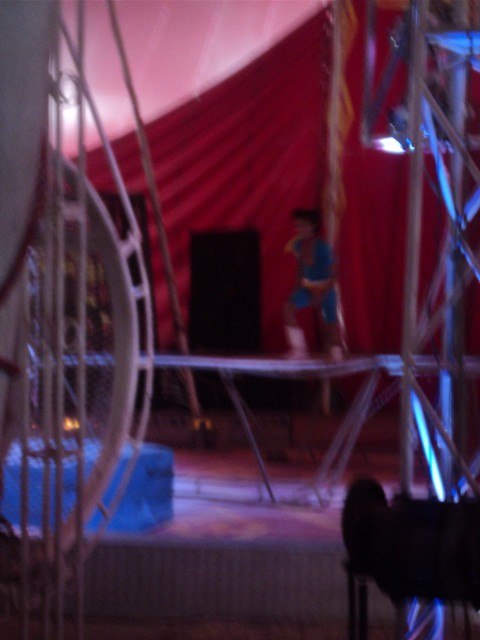The photograph is extremely blurry and grainy, making it difficult to discern precise details. In the background, there appears to be a red tent, potentially indicative of a circus setting. The tent features a couple of rectangular openings or doors and is accented with draped fabric of a lighter color overhead. On both the left and right sides of the image, metal bars or scaffolding are visible, adding to the impression of a structured event space such as a circus or carnival. 

In the distance, a person is seen standing, running, or performing on what might be a trampoline, walking platform, or bridge. This individual appears to be dressed in a blue and red outfit, reminiscent of a superhero costume, possibly similar to a Superman costume, and they are also wearing white boots. A blue plastic tub or mat is positioned on the ground to the left side of the scene, contributing to the array of colorful elements—red, blue, pink, white, silver, and black shadows. The setting is illuminated by various lights, suggesting an event or performance; however, due to the poor image quality, these details remain largely speculative. The photo was likely taken by someone in the audience from some distance away, capturing what seems to be a solitary figure performing amidst a circus-like backdrop.